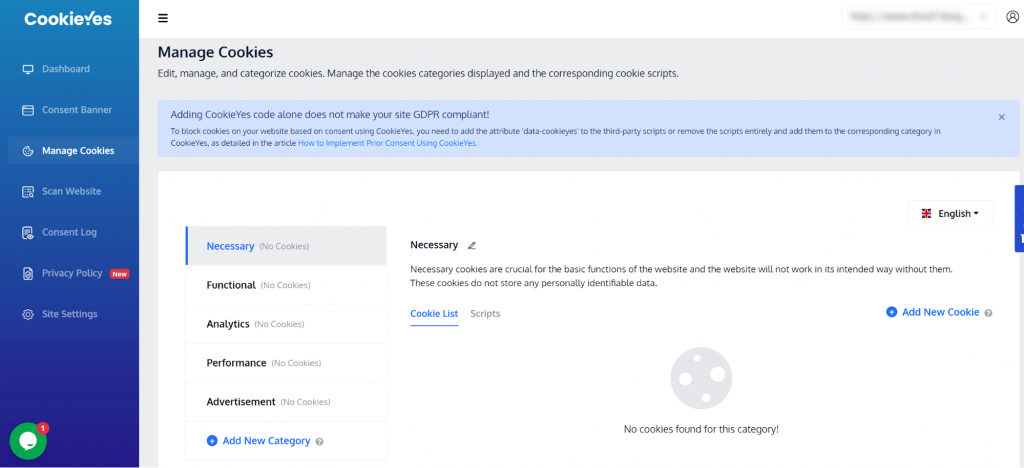This image is a detailed screenshot of a website interface. On the left side, there is a vertical blue rectangle featuring a gradient from lighter blue at the top to darker blue at the bottom. The top of this rectangle displays the text "Cookie Eyes" in white font, where the 'Y' in "Eyes" is stylized as a checkmark. Directly beneath is a vertical menu with options listed in white font: Dashboard, Consent Banner, Manage Cookies, Scan Website, Consent Log, Privacy Policy, and Site Settings. The "Manage Cookies" option is currently selected.

In the lower-left corner of the screen, there is a red circle containing a white chat bubble icon. A smaller red circle positioned in the upper right corner of this chat bubble icon indicates a notification with the number "1".

To the right of this menu, the interface displays the "Manage Cookies" settings section. At the top of this section is a gray rectangle with black font, stating: "Manage Cookies, Edit, Manage, and Categorize Cookies, Manage the Cookies, Categories Displayed, and the Corresponding Cookie Scripts." Below this is a blue rectangle with instructions in white font stating: "Adding Cookies, Yes, Code, Alone, Does Not Make Your Site GDPR Compliant! To block cookies on your website based on consent using Cookie Eyes." The overall layout and text emphasize the steps and settings related to cookie management within the website's interface.